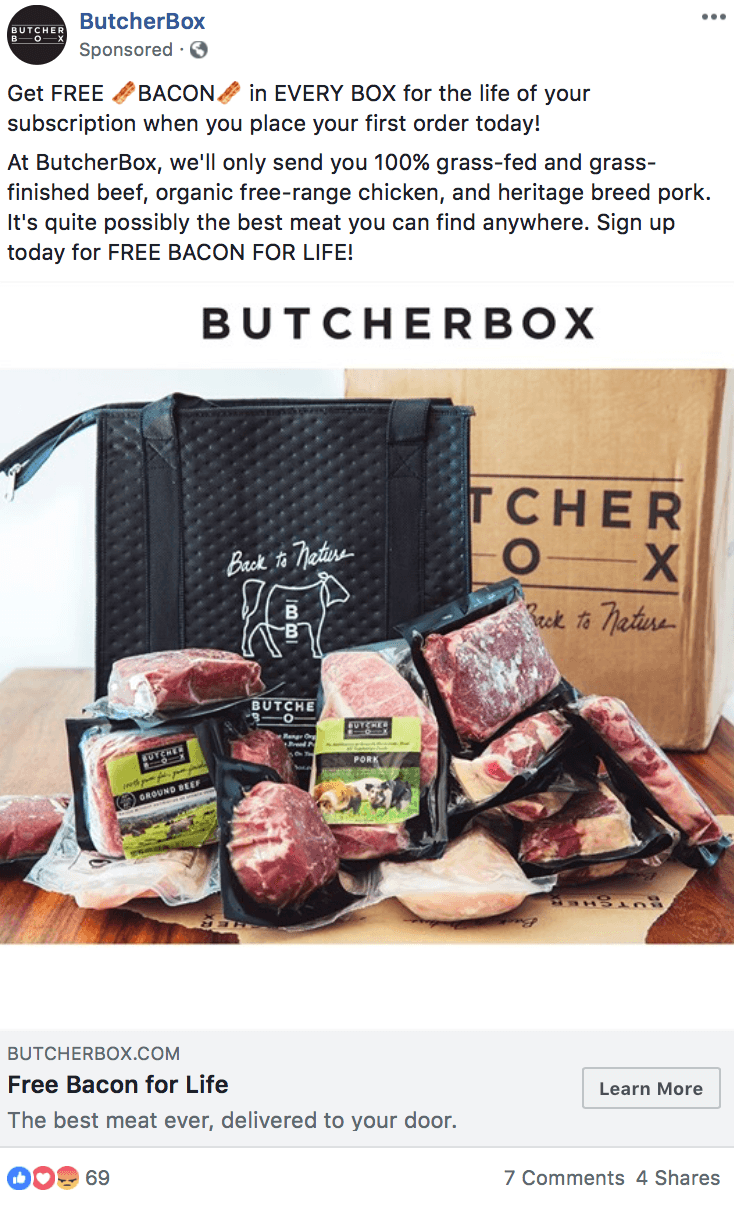This is a screenshot of a sponsored post from the business ButcherBox. The post prominently offers a special promotion: "Get free bacon in every box for the life of your subscription when you place your first order today." The message is followed by a detailed description of the box contents.

At the bottom of the text, in bold capital letters, the brand name "BUTCHERBOX" is displayed. Beneath this, the image showcases various packaged meats arranged artistically on a wooden table. In the background, there's a black tote bag featuring a line drawing of a cow and the phrase "Back to Nature." Additionally, what appears to be a paper grocery bag with the "ButcherBox" logo and "Back to Nature" slogan is visible.

Underneath the image, further promotional text states: "Free bacon for life, the best meat ever delivered to your door." A "Learn More" button is included, showing interactions with the post: 69 reactions (likes, hearts, or other), 7 comments, and 4 shares.